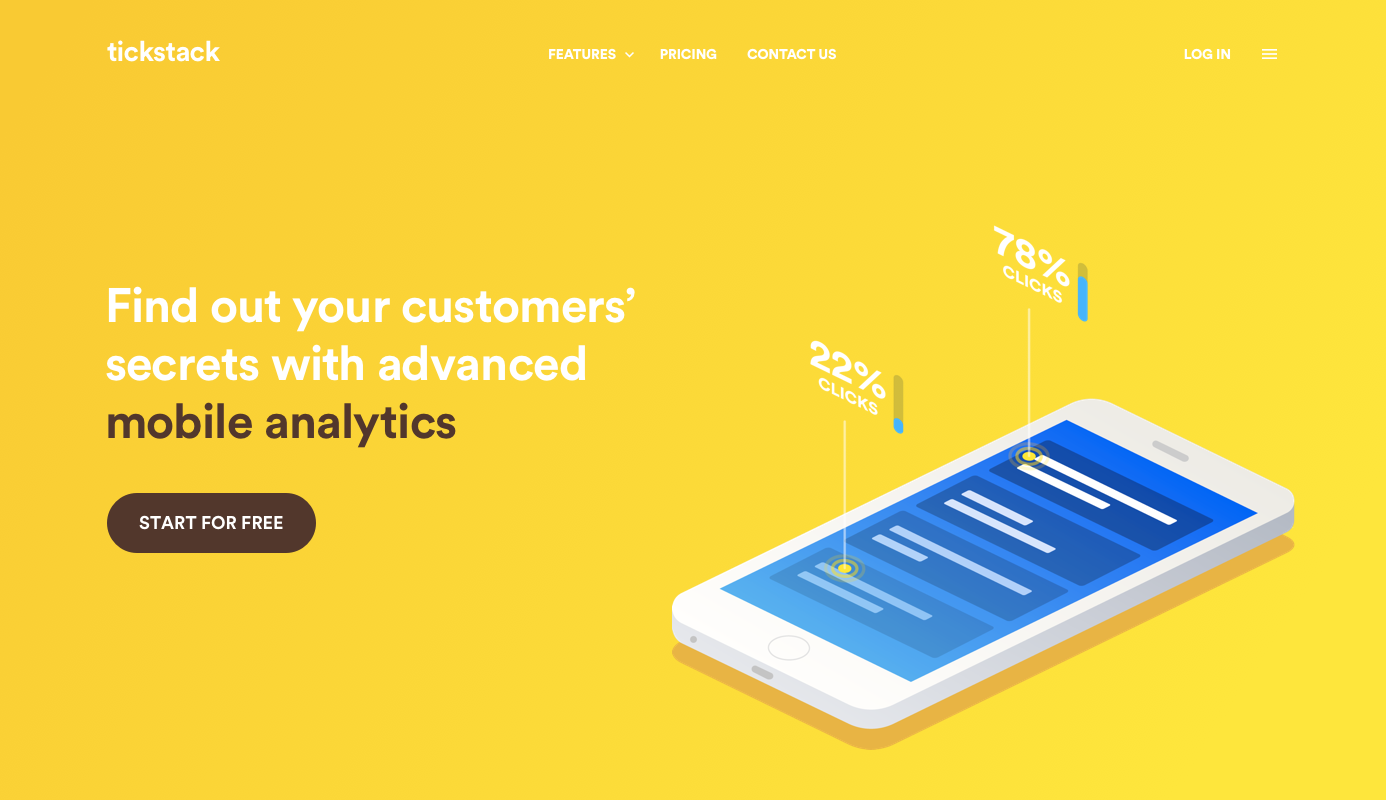The web page features a striking design with a predominantly yellow background that transitions to a darker yellow at the top. On the top left corner, the brand name "Tickstack" is displayed in bold white text. At the top center, navigation options are arranged horizontally: "Features" with a drop-down menu, "Pricing," and "Contact Us." On the top right, there is a "Login" button next to a menu icon represented by three white lines.

Dominating the left side of the page, a bold white headline reads, "Find out your customers' secrets with advanced," followed by the phrase "Mobile Analytics" in a dark brown color. Directly below this text is a clickable, dark brown oval button that invites users to "Start for free" in white text.

On the right-hand side of the screen, there is an image of a smartphone laid flat against a blue background. The smartphone display features several white horizontal bars representing text, accompanied by a yellow dot next to some of these bars. From the topmost yellow dot, a white line extends upward, indicating "78% clicks," accompanied by a blue bar. A second yellow dot lower on the screen also has a white line extending upward, showing "22% clicks," with its respective blue bar.

This detailed layout combines vibrant colors and clear typography to effectively convey the purpose of the web page and its key features.